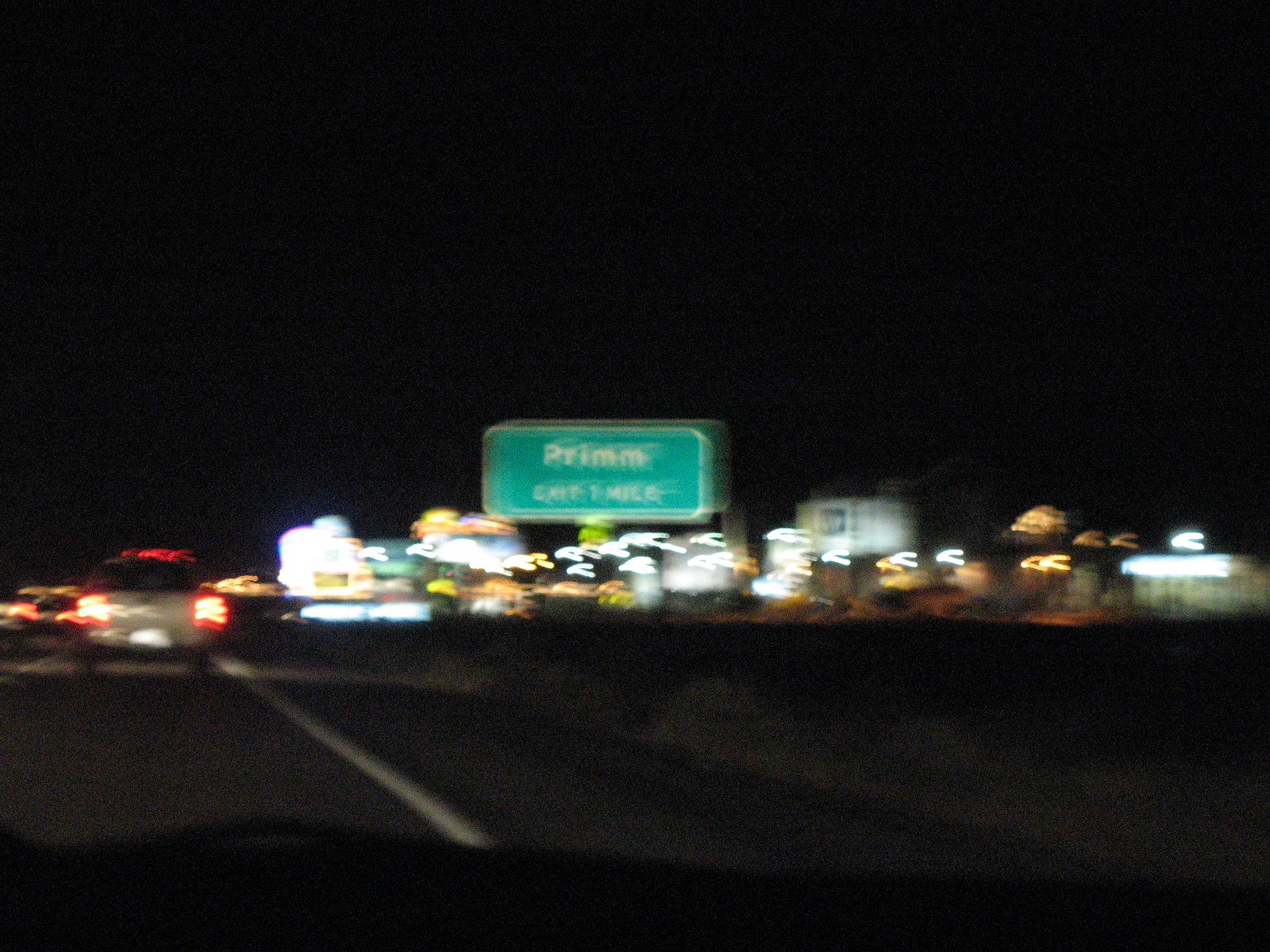This nighttime photograph, taken through a car's front window, captures a blurry urban scene with a distinct green highway sign in the center, reading "PRIMM, P-R-I-M-M, exit one mile." The roadway enters from the lower left, leading towards a white truck visible in the distance, its taillights prominent. The sky and landscape are enveloped in pitch-black darkness, accentuating the illuminated buildings stretching from the center to the right edge, suggesting a town ahead, likely Primm, Nevada. Despite the image's blurriness, the bright neon lights of these structures stand out vividly against the night.